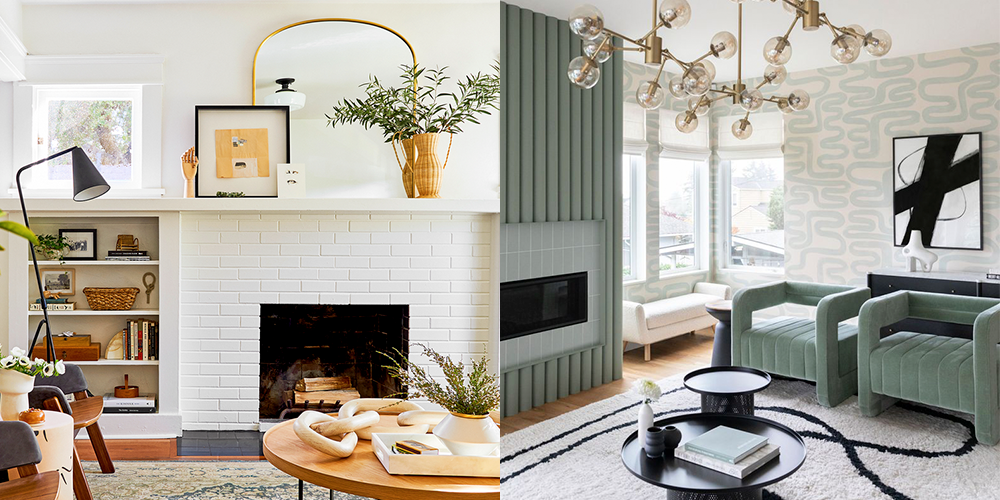The image captures two adjacent rooms, each exemplifying distinct design styles. 

On the left, we observe a mid-century Scandinavian-style room characterized by its white walls, softwood accents, and black industrial decorative elements. Central to this room is a white-painted brick fireplace with a gray trim at the base, above which sits a black-rimmed painting alongside a vase with plants. To the left of the fireplace, there is a built-in bookshelf adorned with woven baskets and books. A circular wooden coffee table and a lamp resembling those found in offices complete the scene, while a pot of flowers adds a touch of natural beauty.

The room on the right embodies a mid-century romantic luxury charm, featuring soft sage accents and a visually striking circular-bulb chandelier with glass globes and gold tubing. This space is revealed to have a teal-painted wall with a modern gas fireplace showcasing a glass front. A small circular metal table with books, a white rug with black lines, and cushioned chairs beneath large, hazy windows enhance the luxurious feel. The transition from the left to the right room highlights a sense of cohesiveness in design evolution, from Scandinavian simplicity to romantic luxury.